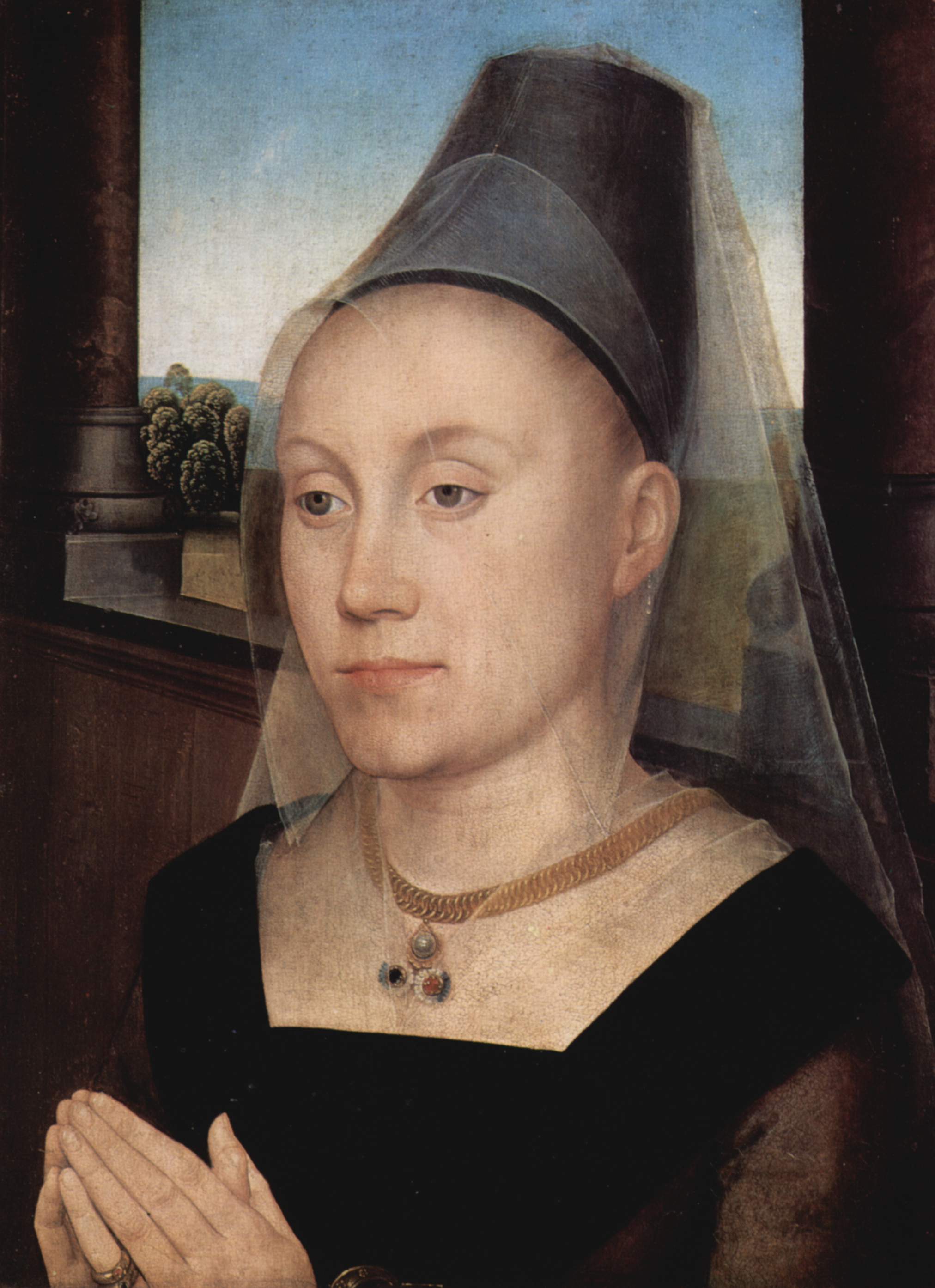This painting is a detailed and realistic portrait of a woman with very fair skin, hazel eyes, and a serene expression as she gazes to the left. She wears a tall black hat with a veil that drapes down the back and subtly covers her face with a netting. Her attire includes a black dress that exposes her shoulders and chest, and a gold or copper necklace with three hanging beads or jewels in red, black, and white or silver. Her hands are clasped together in a prayer position, positioned near the bottom left corner of the painting. She sits against a window with a brown wooden frame, offering a view of the blue sky, a cactus, and blue water outside. The interior features brown wooden walls and dark wooden columns that could suggest a balcony setting or a bench.